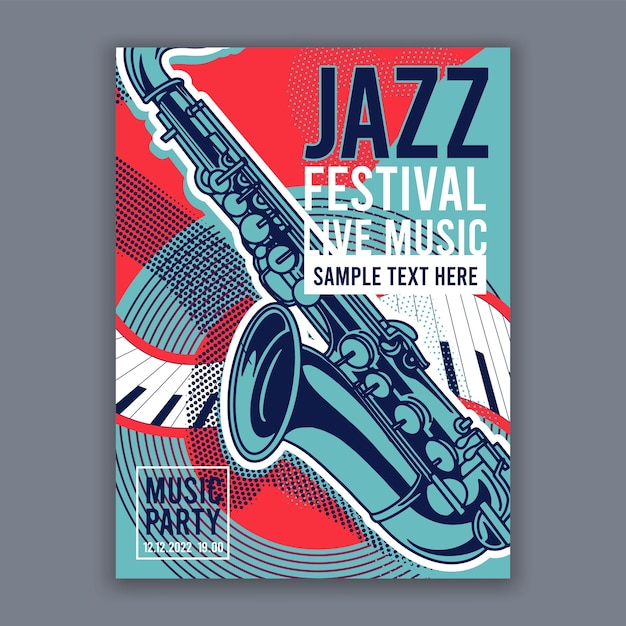The image depicts a detailed close-up digital scan of a jazz festival poster set against a gray-blue background. The poster features a dynamic color scheme predominantly in red and light blue. At the top right corner, the word "JAZZ" is prominently displayed in dark ultramarine blue text, followed by "FESTIVAL" in white text just below, and "LIVE MUSIC" beneath that. Below the phrase "LIVE MUSIC," there is a white rectangle with "SAMPLE TEXT HERE" in navy blue font. Diagonally across the poster, a teal saxophone with navy blue accents is positioned at a 45-degree angle to the left, spanning from the center hole just above the bottom center. Additional design elements include a white keyboard with black keys in the background and concentric circular, purple-toned swirls. In the bottom left corner, inside a transparent box with a white border, the phrase "MUSIC PARTY" is written in blue text, with "12.12.2022, 19:00," displayed just below in white font.